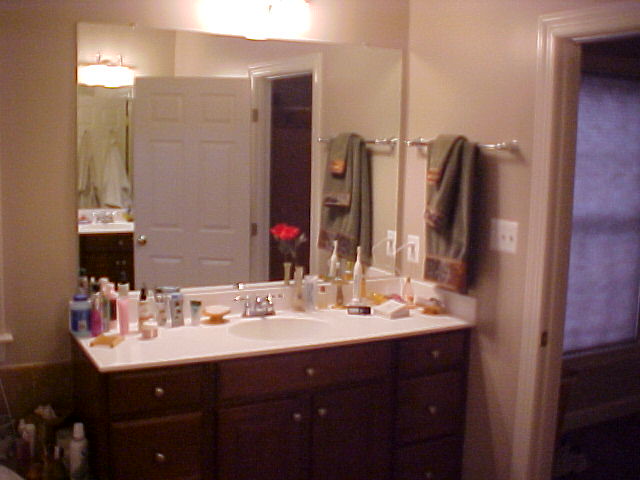A well-lit photograph captures the cozy ambiance of a bathroom at night within a home. The image features a snug corner where the bottom left showcases the edge of a bathtub adorned with various bottles on its surface and partly tiled wall. Ascending from the bathtub, the wall transitions to a calming beige or cream paint. Dominating the scene is a pristine white vanity unit with an integrated sink and multiple drawers and cupboards, complemented by a sleek mixer tap over an oval basin. Above the sink, a large mirror spans the majority of the back wall, topped by a light fixture illuminating the space.

To the right of the basin, a wall-mounted towel rack holds a large towel, a hand towel, and a face towel, providing ample drying options. Adjacent to the towel rack are white light switches positioned next to a door frame on the far right side of the image. Through the door frame, closed curtains suggest a source of light from outside the room.

The vanity counter is dotted with various beauty products, soaps, and a rechargeable toothbrush plugged into a power outlet on the wall. A small vase with a single red rose adds a touch of elegance and color, positioned thoughtfully to the right of the taps. A faint reflection in the mirror hints at a nearby shower or possibly an additional mirror, contributing to the room's reflective ambiance.